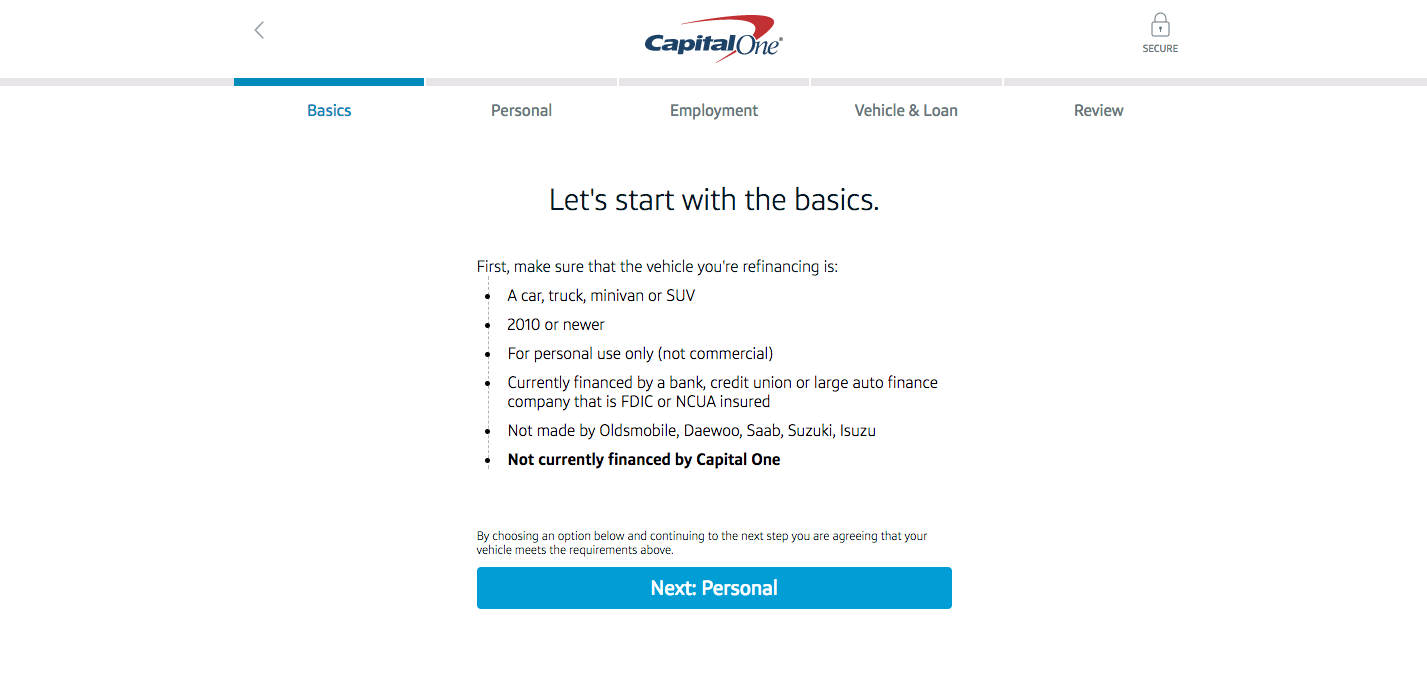This is a detailed screenshot of the Capital One mobile website viewed in landscape mode on a smartphone or tablet, designed to guide users through the vehicle refinancing process. At the top center, the Capital One logo is prominently displayed. On the far left, near the edge of the screen, there's a gray arrow for navigation to go back. On the far right, a small lock icon labeled "secure" assures users that the connection is encrypted.

Below the header, there is a step-by-step navigation bar outlining the stages of the process: Basics, Personal, Employment, Vehicle and Loan, and Review. Currently, the "Basics" step is highlighted in blue, indicating that it is the active section.

In the main content area, the website prompts users with the message, "Let's start with the basics." It then specifies the criteria for the vehicle refinancing: the vehicle must be a car, truck, minivan, or SUV from the year 2010 or newer, intended for personal use, and currently financed by a bank, credit union, or large auto finance company that is FDIC or NCUA insured. The vehicle should not be manufactured by Oldsmobile, Daewoo, Saab, Suzuki, or Isuzu, and it should not be currently financed by Capital One.

At the bottom of this section, there is an option to proceed to the next step labeled "Personal."